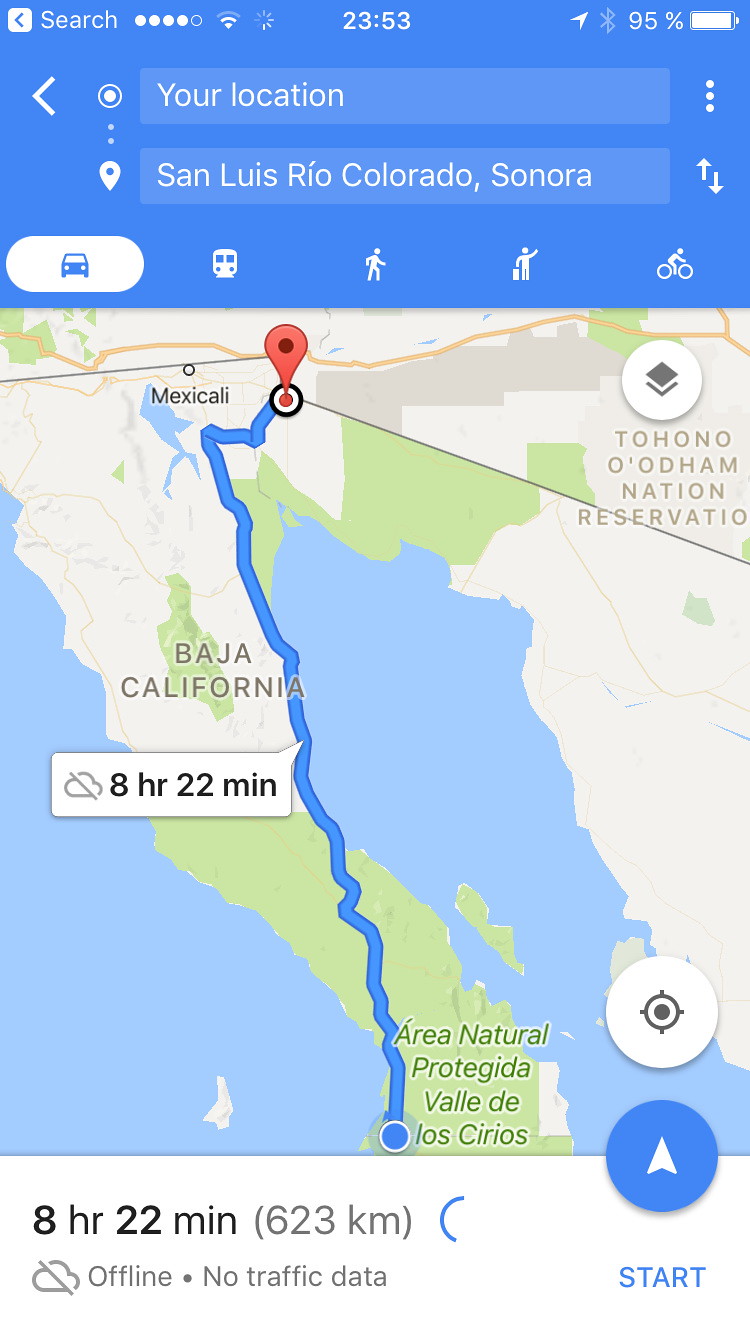The image is a detailed screenshot of a Google Maps navigation route displayed on a mobile phone screen. The top of the screen features standard phone indicators such as the battery level at 95%, Wi-Fi and cell signal icons, and the time displayed in military format (23:53). The Google Maps interface shows a thick blue border at the top and a thinner white border at the bottom. 

The map itself details a long route by car, estimating an 8 hour and 22-minute journey covering 623 kilometers. The starting point is near Baja California and the final destination is San Luis Rio Colorado, Sonora, situated towards the southern tip. The image also indicates that the map is currently offline, as shown by a small cloud icon with a cross through it.

Additionally, the maps image includes a search bar at the top and a blue "Start" button for the navigation at the bottom right corner of the screen. There's also an option to see the current location zoomed in. Other visible elements include a Bluetooth symbol and various map colors like blue, green, and tan to indicate different terrains and features of the route.